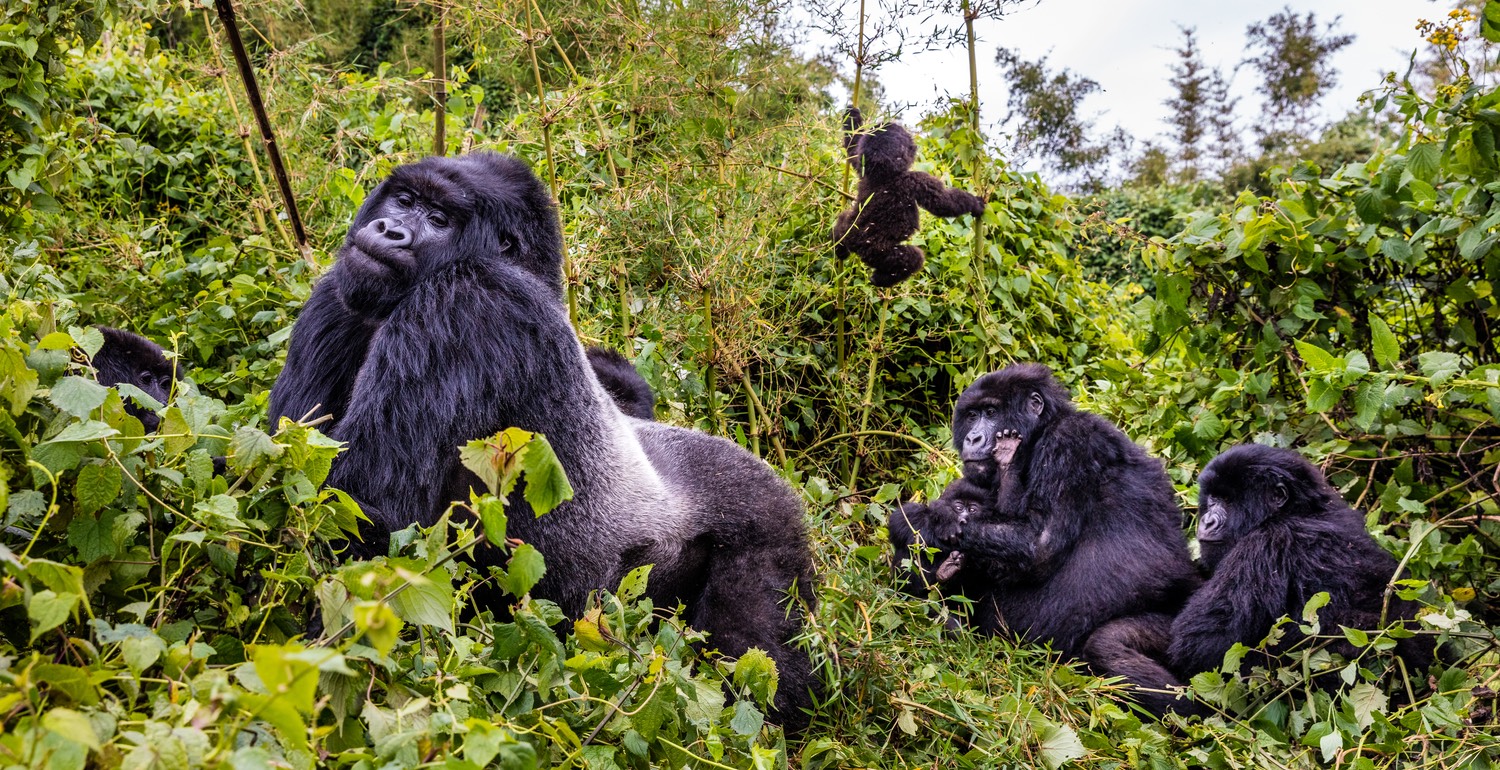This color photograph, reminiscent of a scene from a National Geographic magazine, captures six gorillas in a lush, overgrown forest field, blanketed with shrubs, vines, and grasses. Dominating the foreground is a large, majestic silver-backed male gorilla on all fours, with an arched back and his head slightly tilted towards the camera, showcasing his distinct black shaggy fur and silver back. In front of him, partially obscured by foliage, are the eyes and the top of the head of a small gorilla. Behind the silverback, another gorilla is seated, facing the larger one and cradling a baby gorilla, which grips its mother's arm with one hand while reaching towards her face with the other. Adjacent to them, another similarly sized gorilla sits, and at the bottom right of the image, a smaller gorilla is visible. In the background, high up among the leafy greenery, a playful baby gorilla grips two tree stalks, swinging between the branches in a picturesque display of the natural world. A sliver of blue sky peeks through the upper right corner, adding a serene backdrop to this captivating scene of gorilla family dynamics.